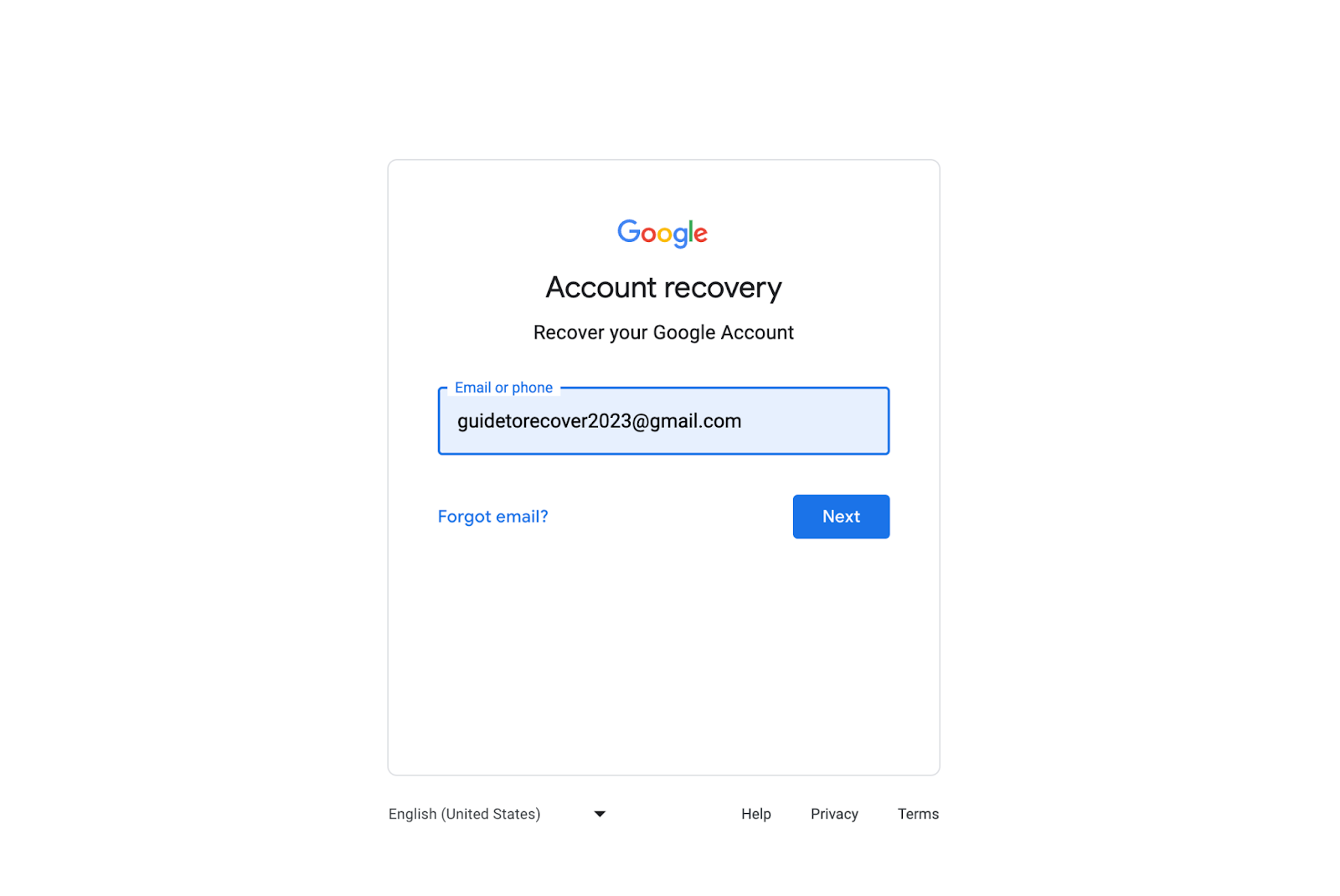The image appears to be a screenshot taken from a phone or a website, featuring a Google account recovery page. The background is predominantly white with a box outlined by a thin gray line centered on the page. 

At the top of this box, the Google logo is displayed prominently. The logo features the iconic multi-colored letters, with the first "G" in blue, followed by "o" in red, "o" in yellow, "g" in blue, "l" in green, and "e" in red. The first "G" is capitalized, while the rest of the letters are in lowercase.

Beneath the logo, bold black text reads: "Accounts Recovery," with only the "A" capitalized. Following this, there is another line of text in black that says: "Recover Your Google Account," where "Recover," "Google," and "Account" are capitalized.

Further down, a search bar is highlighted by a thin blue line and filled with a lighter shade of blue, indicating it is active. Inside this bar, on the top left, blue text reads: "Email or Phone." Below this, in black text, an email address is visible: "guidetorecover2023@gmail.com," all in lowercase.

To the left of this bar, in blue text, is the option: "Forgot email?" To the right of this bar is a dark blue button with white lettering that says "Next."

At the bottom of the box, aligned to the left, black text reads: "English (United States)" with a drop-down arrow indicating selectable options. On the bottom-right corner, three black text links read: "Help," "Privacy," and "Terms."